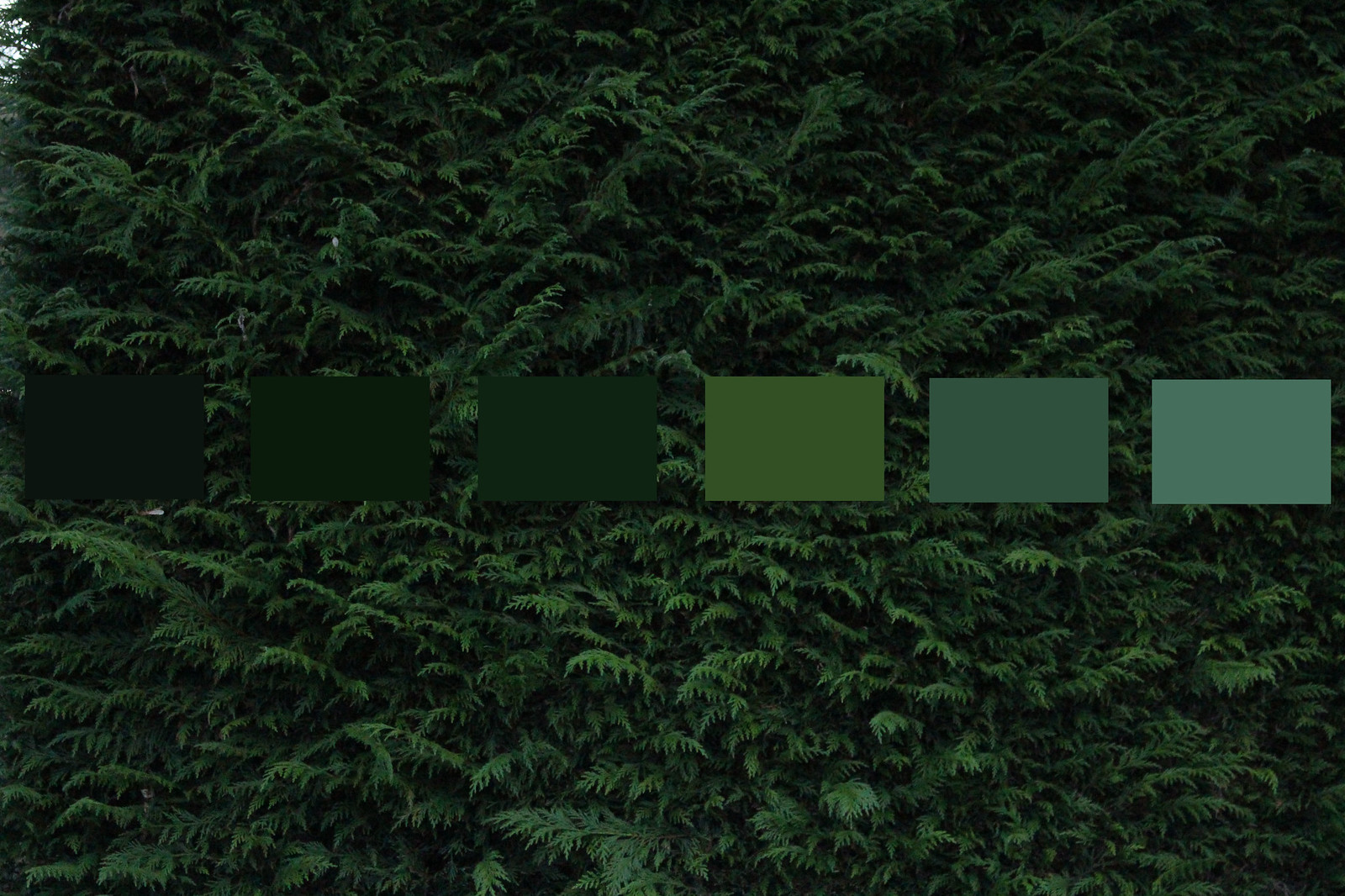This photograph captures the deep green foliage of an evergreen tree, filling the entire frame with its needle-like leaves. The image features an overlaid color gradient composed of six rectangular shades of green, arranged from left to right. Starting on the left, the gradient transitions from a very dark, nearly black green to a pastel green on the right. The color palette includes shades such as forest green and olive green, providing a comprehensive range of green hues present in the foliage. The lighting is subdued, suggesting the photo might have been taken outdoors on an overcast day, adding to the overall natural ambiance.